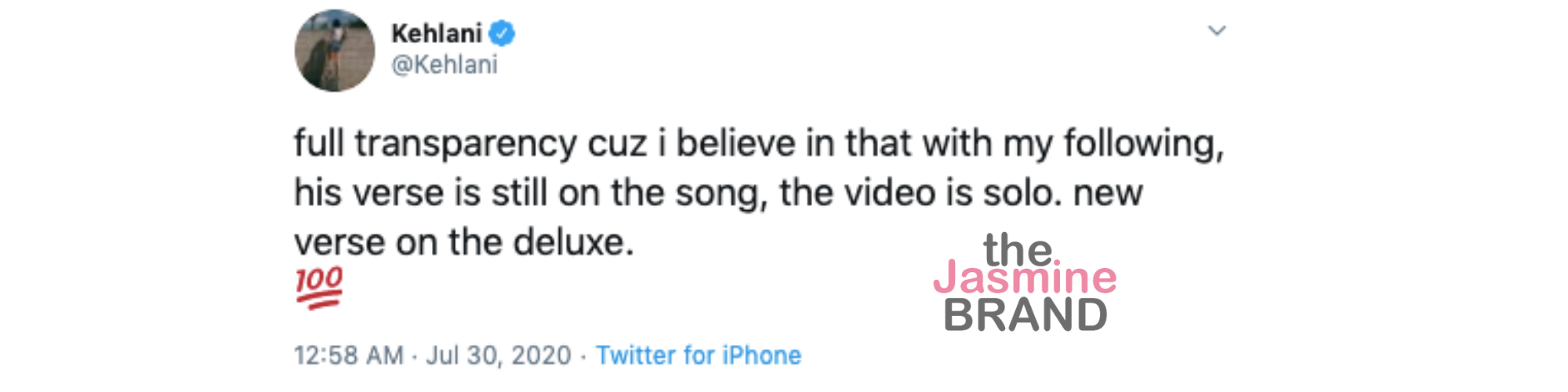This is a screenshot of a tweet featuring a white background with predominantly black text. In the top left corner, there is a circular profile photo of the user. Beside it, "Kehlani" is written in bold black font, followed by a blue verified badge—a blue circle with a white check mark inside. Below this, the user's handle "@Kehlani" is displayed.

The main content of the tweet is presented in all lowercase and reads: "full transparency cuz i believe in that with my following, his verse is still on the song, the video is solo, new verse on the deluxe." Following the text, there is a red "100" emoji with two red lines beneath it.

On the far right side of the tweet, an additional annotation reads "The Jasmine Brand," with "Jasmine" highlighted in pink. At the bottom of the tweet, the timestamp "12:58 AM · Jul 30, 2020" is shown, followed by "Twitter for iPhone" in blue text.